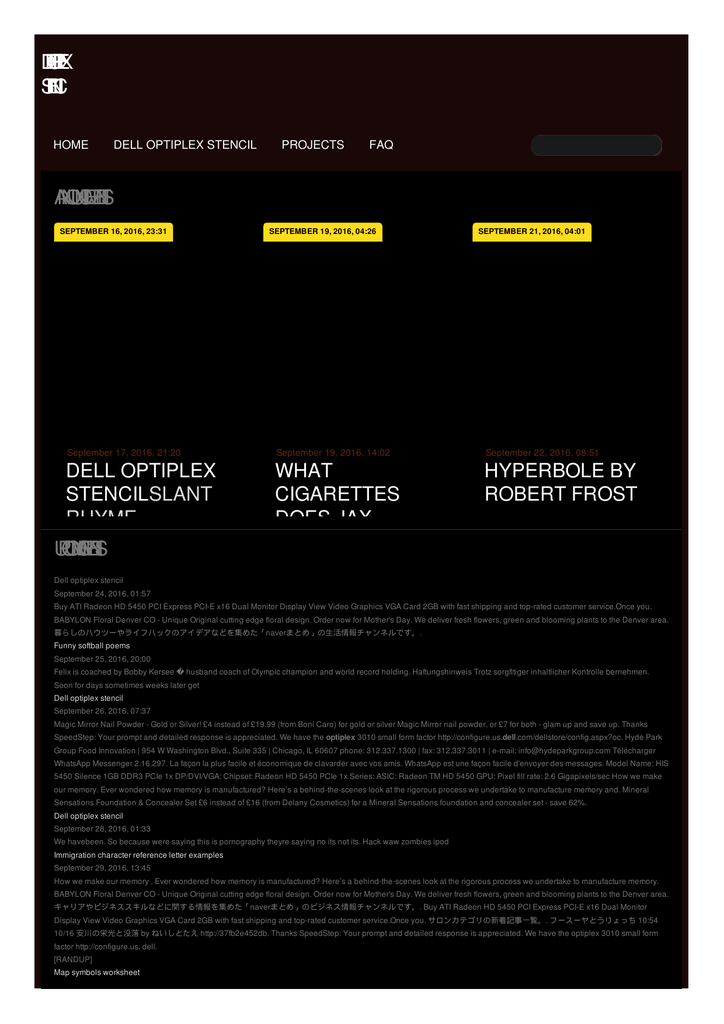The image is a screenshot showcasing a user interface with a dark reddish-brown bar at the top. In the top left corner, partially overlaid letters "S" and "C" are visible, mostly obscured by one another. To the right of these letters, a white menu bar stretches horizontally, featuring the options: "Home," "Dell Optiplex Stencil," "Projects," and "FAQ."

Directly below the menu bar are three rectangular buttons with slightly rounded edges, each displaying a timestamp. The first button features black text reading, "September 16, 2016, 23:31." The second button is marked with "September 19, 2016, 04:26," while the third button shows "September 21, 2016, 04:01."

Further down in the screenshot, three lines of prominent white text are listed, each corresponding to a piece of content or title and prefaced by a date and time. The first line reads, "Dell Optiplex Stencil Slant," with a timestamp above it stating, "September 17, 2016, 21:20." The second line declares, "What Cigarettes?" accompanied by the timestamp, "September 19, 2016, 14:02." The final line displays, "Hyperbole by Robert Frost," with the corresponding time, "September 22, 2016, 08:51."